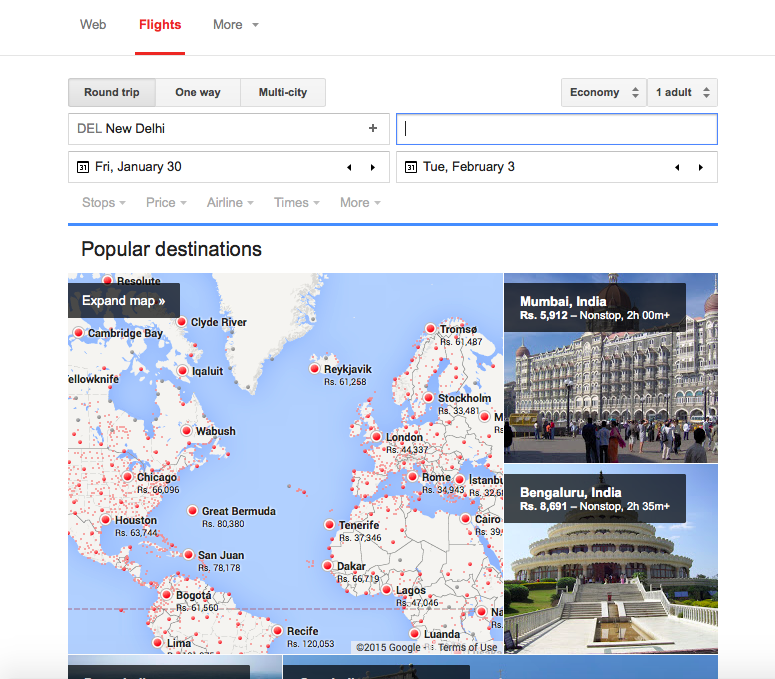The webpage features a user interface of a travel booking website. In the upper left corner, there are three navigational menu options: "Web," "Flights" (highlighted and underlined in red), and "More." Directly below these options, there are selections for different types of trips, including "Round Trip," "One Way," and "Multi-City," all written in black text.

The map dominates the center to the bottom of the page, displaying various cities marked with small red dots and circles. Blue areas on the map represent bodies of water such as oceans and seas.

To the right side of the webpage, there are two smaller, square-framed images. The upper image shows a large, multi-story gray building and is labeled "Mumbai, India." Underneath, there is additional information: "5,912 non-stop, 2 hours 00 minutes plus."